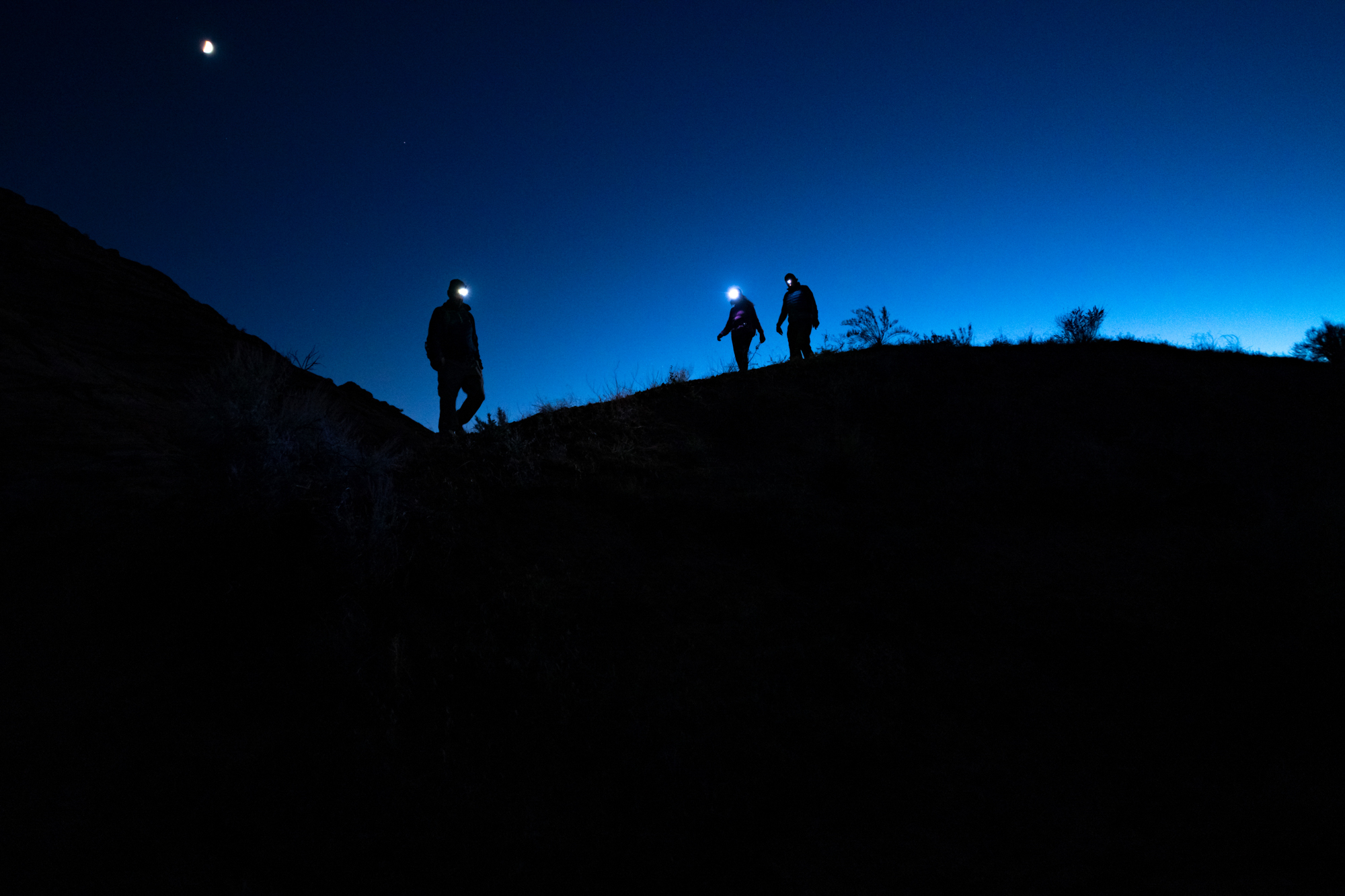The photograph captures a striking nighttime scene of three individuals silhouetted against a dark, hilly landscape. Each person is wearing a headlamp that casts a bright white light, creating eerie yet captivating reflections. The figure positioned to the left is illuminated the most, with a pronounced light near the head. The middle figure also has a noticeable headlamp glow, while the person on the right is dimly lit by comparison. The terrain is predominantly black, with subtle outlines of scrubby plants and hills undulating from the high left side to a dip before minorly rising again. Above, the sky transitions from a dark gradient in the upper left, featuring a faint white moon, to a lighter blue hue on the right, providing a stark contrast to the black foreground. The immersive nighttime ambiance makes it seem as though the photographer is discreetly observing the scene from a lower vantage point. The overall composition emphasizes the silhouettes of the individuals and their quest-like demeanor, enhancing the mysterious and exploratory feel of the image.